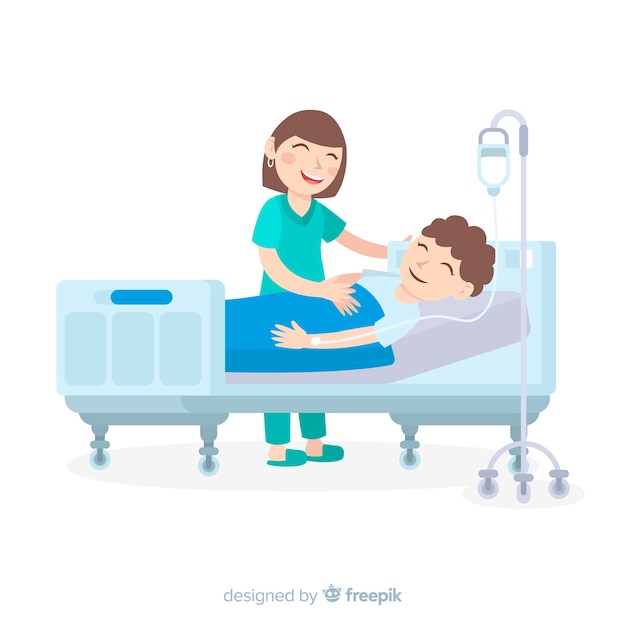The image depicts a colorful, comic-style illustration set in a hospital scene. A nurse with short, straight brown hair, smiling joyfully with closed eyes, is wearing a matching green outfit comprising a nurse’s uniform, pants, and slippers. She's attending to a patient lying in a slightly inclined, light blue hospital bed that has a small fence at the foot. The patient, a boy with brown curly hair and light skin, is under a blue blanket and is also smiling with his eyes closed, exuding happiness. He has an IV tube connected to his wrist, which is attached to a stand placed near the head of the bed. The animated illustration lacks any additional background details, set against the white surface of the screen.